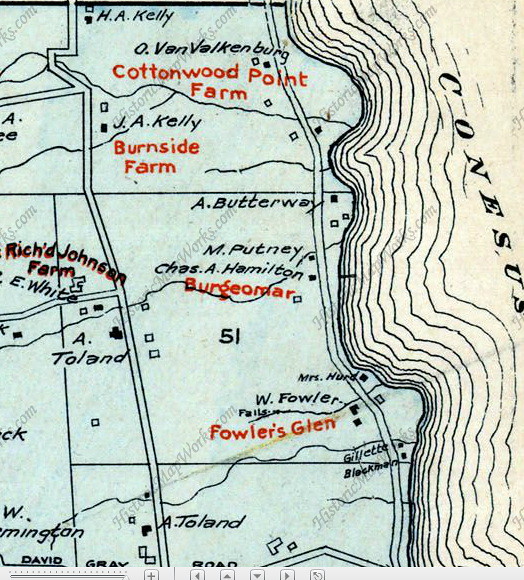This image showcases a detailed, historically styled map, predominantly colored with light blue on the left half and cream on the right half, where the word "Conscious" is prominently written. The map is adorned with various points of interest and names, marked both in black and red text. Notable locations include Cottonwood Point Farm, Burnside Farm, Perjumer, and Owlers Glen. Personal names like H. A. Kelly, J. A. Kelly, A. Butterway, M. Putney, Chasse A. Hamilton, and A. Toland are scattered across the map. The entire image is dominated by the map, which appears hand-drawn and colored, likely with colored pencils, giving it an animated and crafted look. Watermarks reading "historicmapworks.com" are subtly placed throughout the map, adding to its vintage appeal.